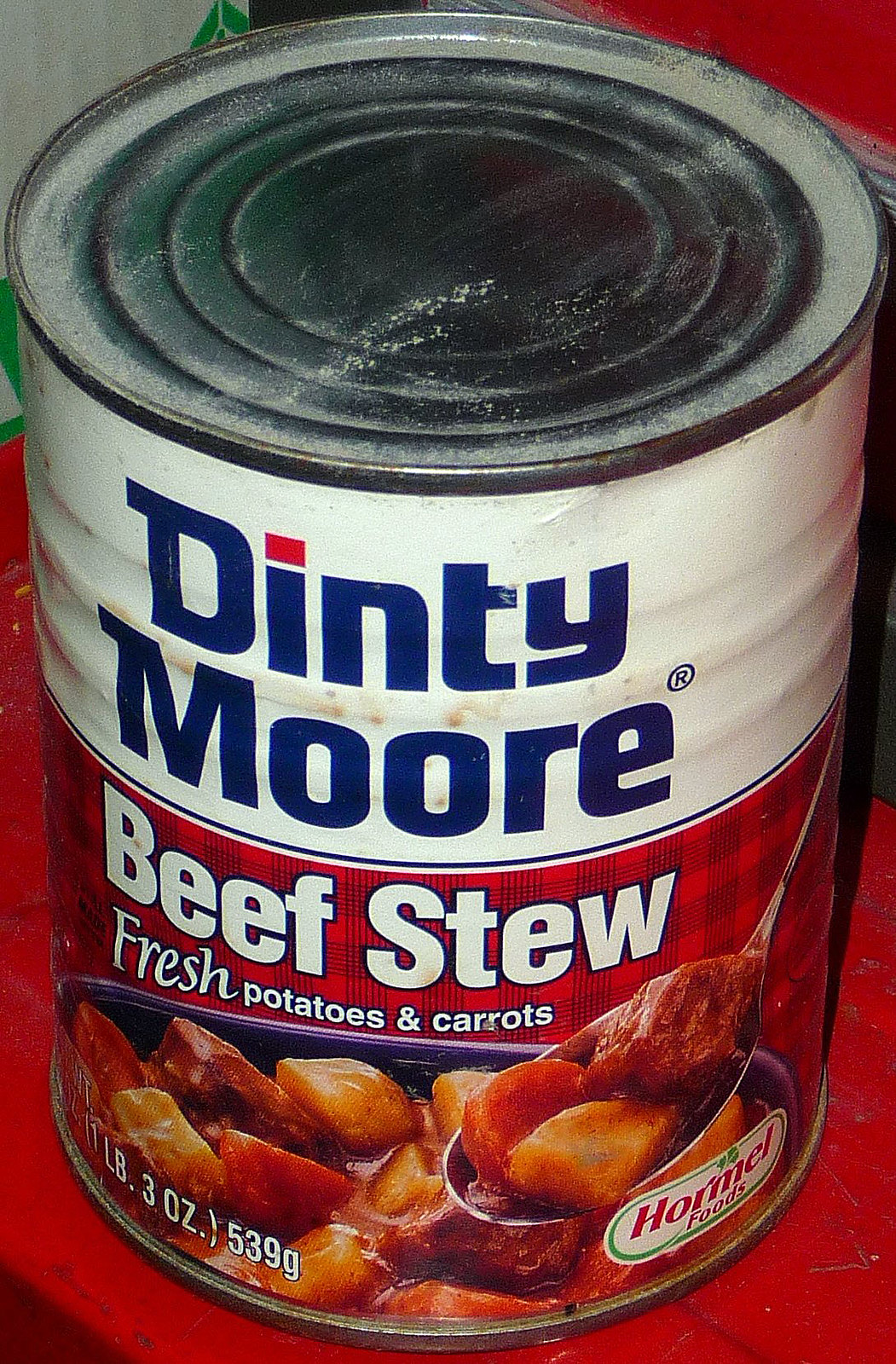The image showcases a can of Dinty Moore beef stew positioned prominently against a mixed red and white backdrop. The can has a silver top with integrated pull-rings for easy opening. The upper section of the can is white, prominently displaying the Dinty Moore logo. Below, the can features a red label adorned with black scratch marks forming a grid-like pattern. The left side of the label reads "Beef Stew," alongside illustrations of fresh potatoes and carrots. The bottom left corner of the label states the weight, "1 lb 3 oz (539 g)." On the right side, a white circle with a green border houses the logo "Horme All Foods." The design within shows a person savoring the beef stew with a spoonful that displays chunks of yellowish potatoes, vibrant orange carrots, and reddish pieces of meat, all immersed in a rich, red-colored sauce.